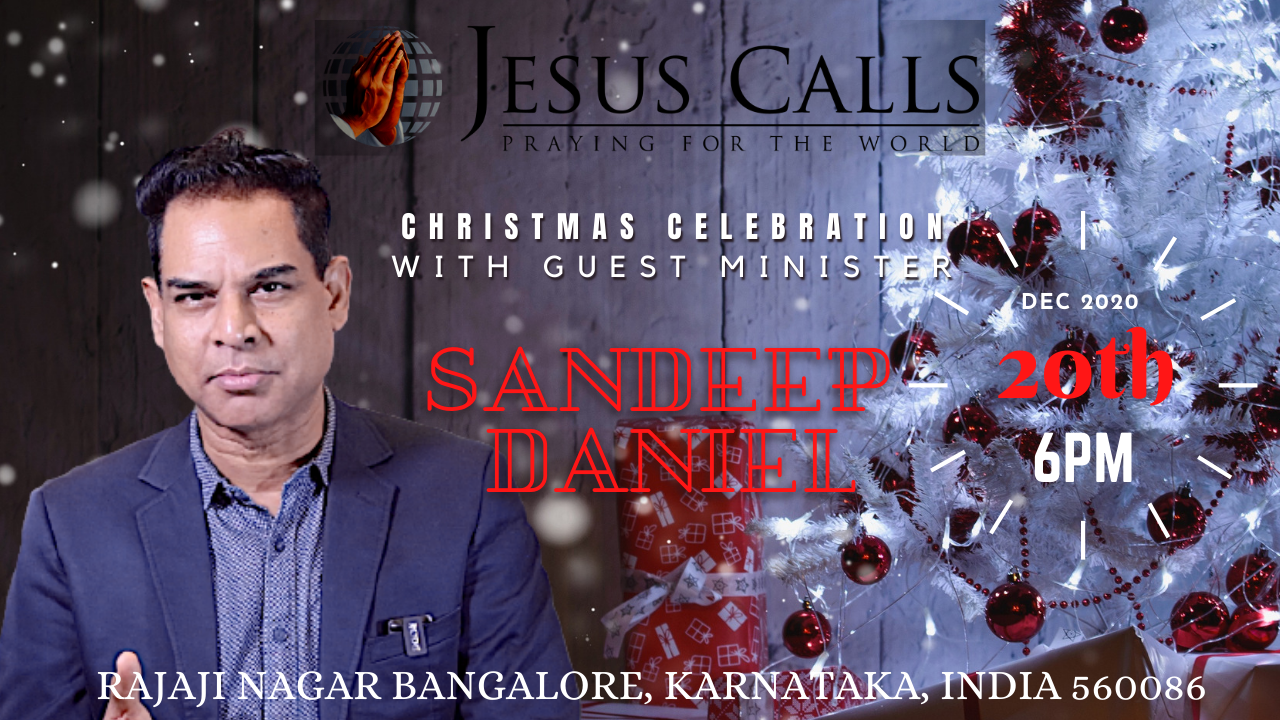This advertisement showcases a religious event organized by Jesus Calls, under the banner "Praying for the World." The background features a whitewashed fence on the left and a white artificial Christmas tree adorned with red bulbs, tinsel, and a red garland on the right. At the top center, large black letters spell out "Jesus Calls," and just below that, a tagline reads "Praying for the World," flanked by a globe with praying hands.

In the middle of the poster, white text announces a "Christmas Celebration with Guest Minister." Prominently displayed beneath in bold red letters is the name "Sandeep Daniel." Further details below this mention the event date "December 20, 2020" and the time "6 p.m." The date and time are creatively depicted within a circular, clock-like design.

On the left side of the image is a photograph of the guest minister, Sandeep Daniel. He is pictured with slicked-back dark hair, a serious expression, and a blue suit jacket over a light blue shirt. He stands with his head slightly cocked, slightly pointing forward with his right hand. The background has a subtle pattern of blue and white dots, enhancing the visual appeal of the poster. The event location is listed as Rajajinagar, Bangalore, Karnataka, India 560086.